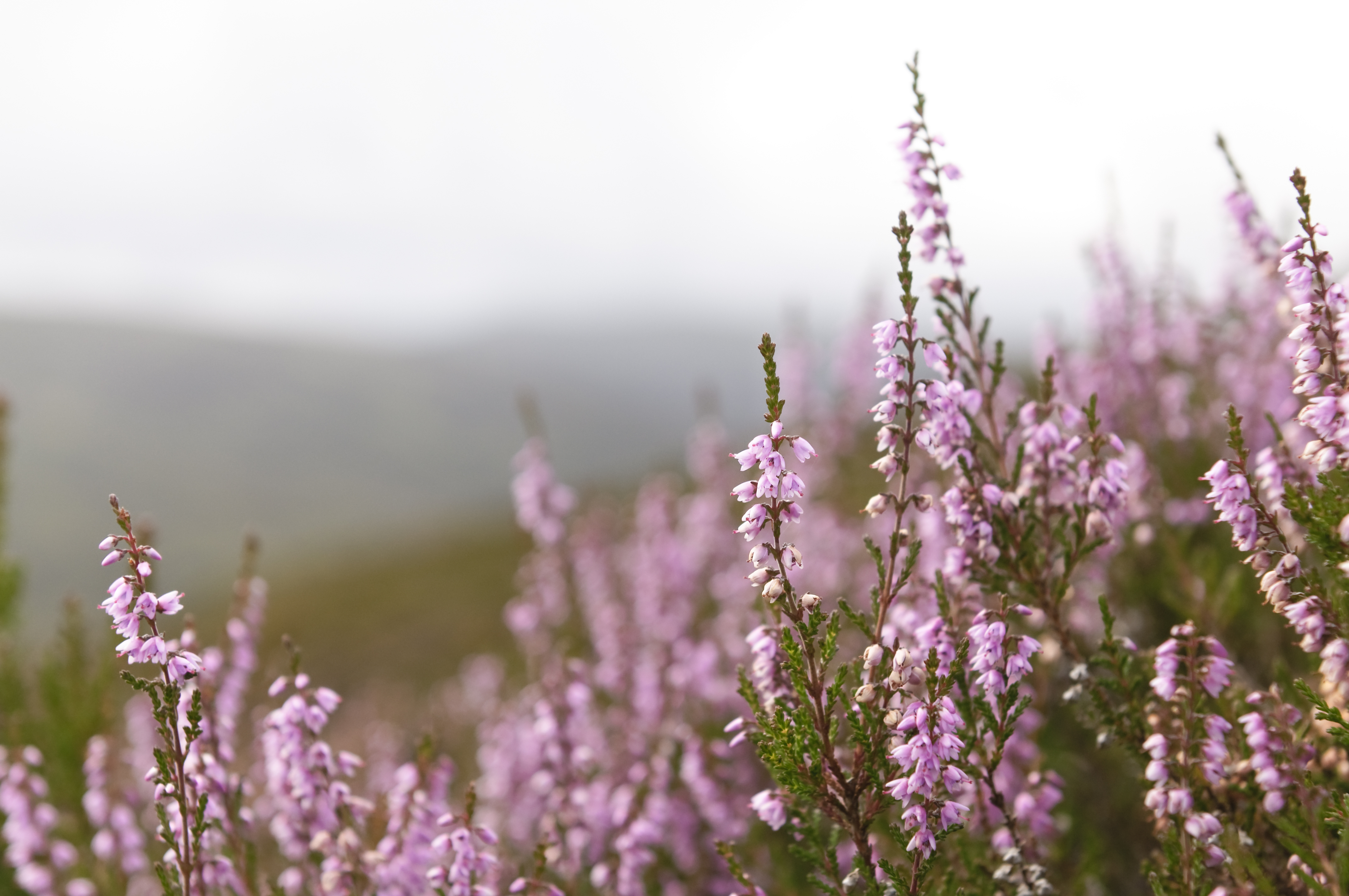This photograph captures the delicate beauty of heather plants in bloom, set against an overcast sky with hills in the distance. The foreground showcases long, slender stems tipped with tiny, pale purple flowers, which have a subtle gradation from white to more pronounced purple hues. The flowers, some shaped almost like bells or trumpets, are meticulously in focus towards the lower right corner of the image, displaying their elegant, cone-like clusters. The greenery of the stems and leaves amplifies the delicate nature of the blossoms, which stand out vividly. As the image recedes, the focus softens, revealing a picturesque, blurred backdrop of rolling hills and a light-colored, cloudy sky that suggests an early spring day. The scene evokes a serene hillside teeming with these elegant, small blossoms that contribute to the overall breathtaking landscape, rich in natural hues and subtle textures.